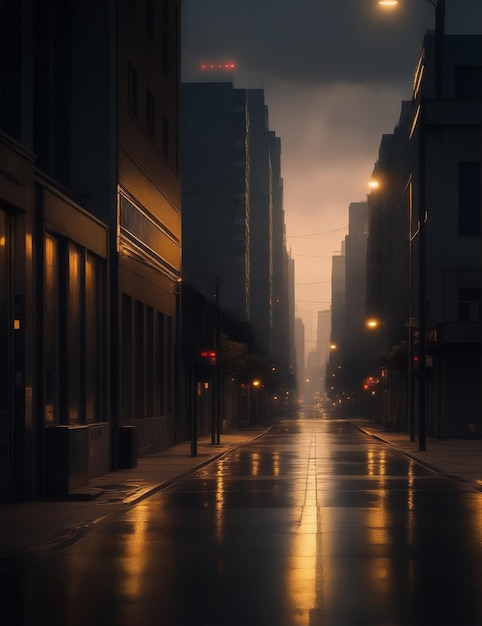The image captures a quiet city street at dusk, viewed from street level and extending straight ahead. Tall buildings line both sides of the two-lane road, creating a corridor of urban architecture. The wet pavement, likely from recent rain, glistens and reflects the numerous streetlights, casting elongated lines of orange and yellow light along the dark, glossy surface of the road. The sidewalks on either side feature additional light posts, trash cans, and a few telephone poles, all devoid of people, suggesting a calm, post-business hours setting. Overhead, wires stretch from building to building, adding to the urban feel, while a solitary red light shines from the top of a distant building. The sky above is gray and cloudy, with the last light of the day fading between the buildings, marking the transition from day to night.